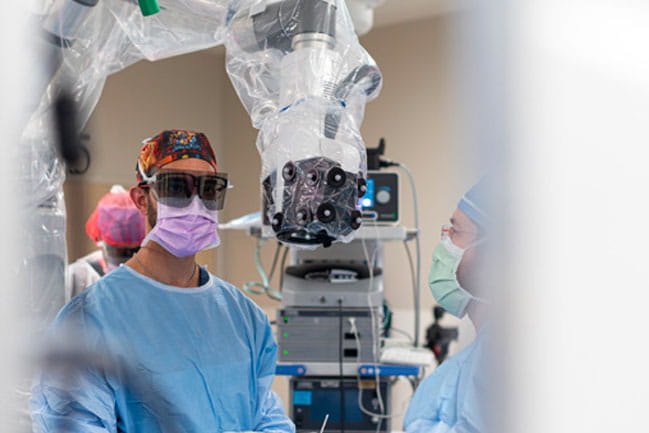This detailed color photograph, captured in a landscape orientation, portrays an active operating room scene with several medical professionals preparing for a surgical procedure. The personnel are all dressed in blue surgical scrubs, masks, and headgear. Notably, one individual on the left is distinguished by a dark gray visor over his eyes and a multicolored skull cap, paired with a pink surgical mask and a blue gown, facing the camera from the top of his head to about mid-chest. To his right, another worker is partially visible in profile, also attired in blue surgical garb.

In the background, the blurred peripheries on the left and right hint at a bustling environment filled with medical equipment. A significant piece of apparatus in the image is an overhead magnifying camera, likely equipped with a microscope for detailed surgical views, encased in clear plastic. This camera is positioned centrally at the top of the photograph, adjacent to a stack of monitors trailing numerous cables, reinforcing the high-tech nature of the setting. The image epitomizes photographic representational realism, capturing the intensity and preparedness of medical professionals in a clinical operating room.